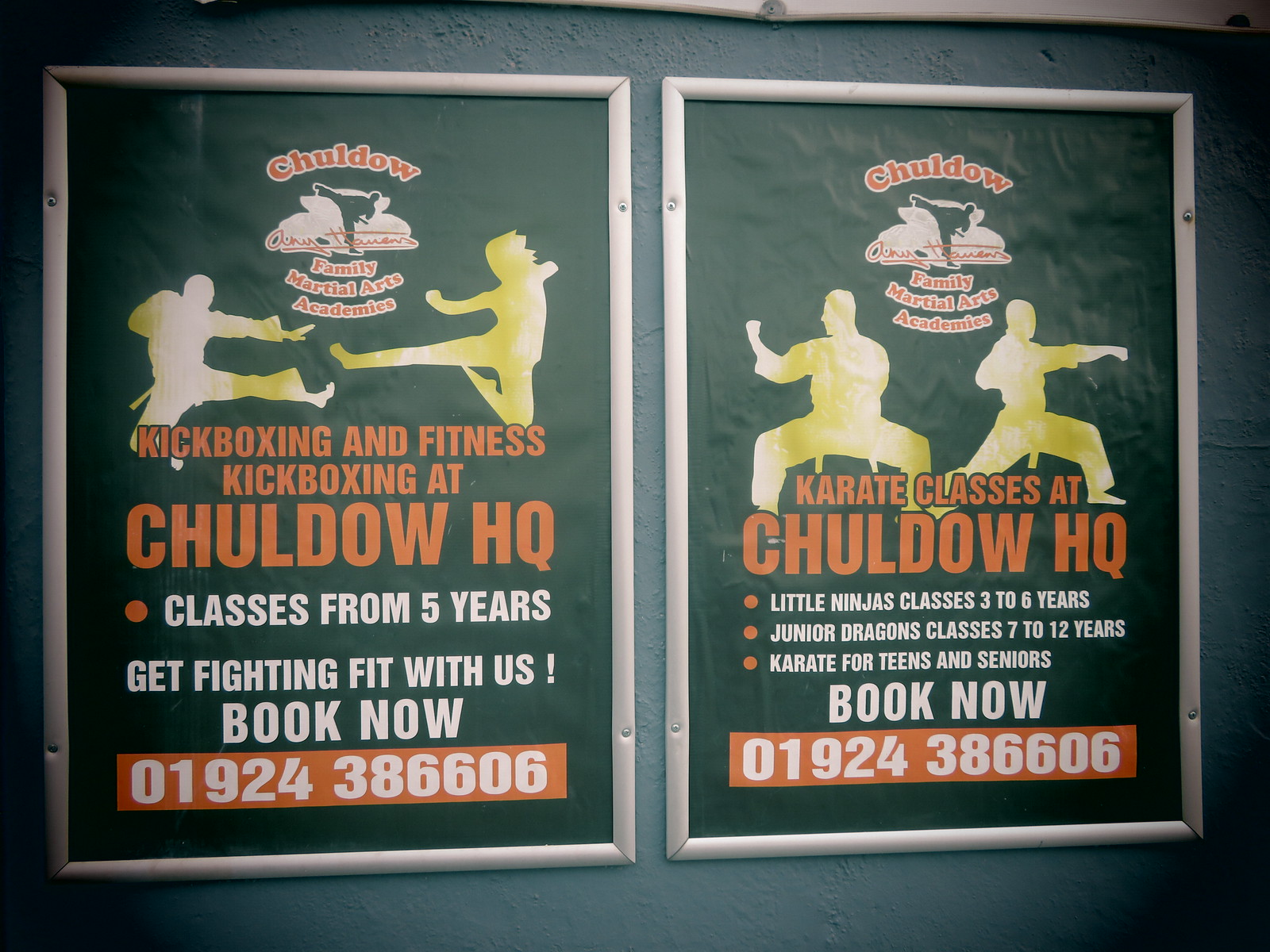Here is a detailed and cleaned-up caption for the advertisement:

---

This advertisement showcases martial arts classes offered by Childo HQ. The design features two distinct images set against a black backdrop, utilizing a striking color palette of red, black, yellow, and white.

The left image promotes kickboxing classes. At the top, the word "Childo" appears, though it's somewhat difficult to decipher. It includes a graphic of two yellow silhouettes engaging in a martial arts move, appearing to kick or punch each other from a distance. Below this graphic, the text reads in bold red lettering, "Kickboxing and Fitness Kickboxing at Childo HQ." Following this, in crisp white letters, the text states, "Classes from five years. Get fighting with us now. Book now." Additionally, a contact code is provided: 01924386606.

To the right, the second image advertises karate classes available at Childo HQ. The specifics include "Little Ninja Classes" for ages 3 to 6 years, "Junior Dragons Classes" for ages 7 to 12 years, and "Karate for Teens and Seniors." It also encourages immediate booking with the phrase "Book now," and lists the same contact code: 01924386606.

Overall, the advertisement vividly highlights the diverse martial arts programs available for different age groups, enticing prospective clients to join and get active.